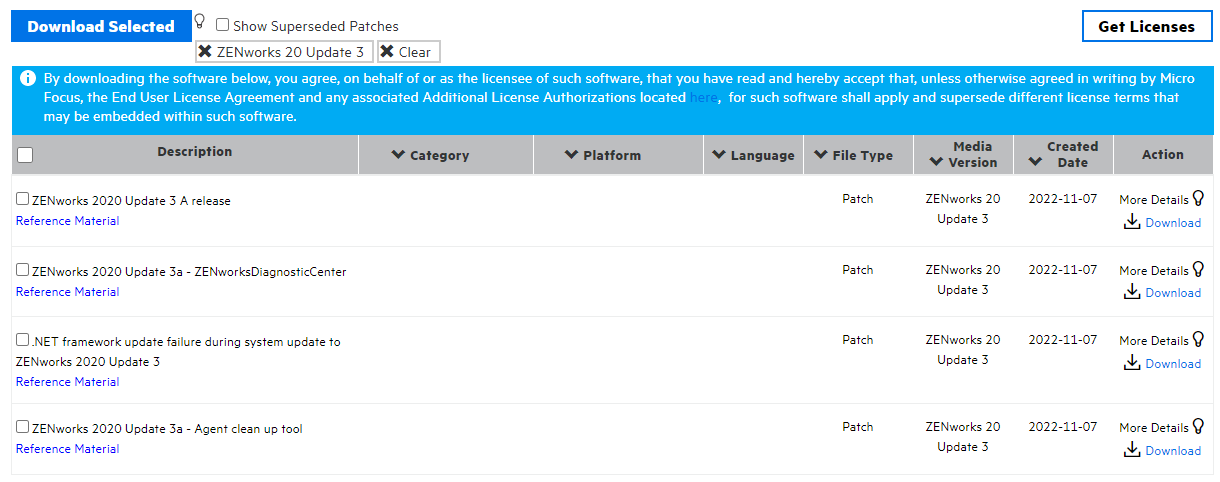The image depicts a computer screen displaying a download interface for software updates. The main content area features a prominent blue button labeled "Download Selected." Below this button, there is a checkbox option labeled "Show Superseded Patches," currently unchecked.

The page is categorized with tags such as "ZENworks 20," "Update 3," and "Clear." Additionally, an informational section begins with an "i" icon, detailing the terms and conditions for downloading the software. It states: "By downloading the software below, you agree on behalf of or as the licensee of such software that you have read and hereby accept that, unless otherwise agreed in writing by Micro Focus, the End User License Agreement and any associated additional license number authorizations located here for such software shall apply and supersede different license terms that may be embedded within such software."

The download section features four distinct options, each classified as a patch:

1. **ZENworks 2020 Update 3a Release**: Accompanied by a button for "Reference Material," it is categorized as Patch Media, version ZENworks 20 Update 3, with a creation date of 2022-11-07.
2. **ZENworks 2020 Update 3a ZENworks Diagnostic Center**: Also classified as a patch.
3. **Dotnet Framework Update Failure During System Update to ZENworks 2020 Update 3**: Categorized as a patch.
4. **ZENworks 2020 Update 3a Agent Cleanup Tool**: Classified as a patch with a creation date of 2022-11-07.

The interface mostly features a white background, with one section highlighted in blue and text in white. Category headings are presented in gray.